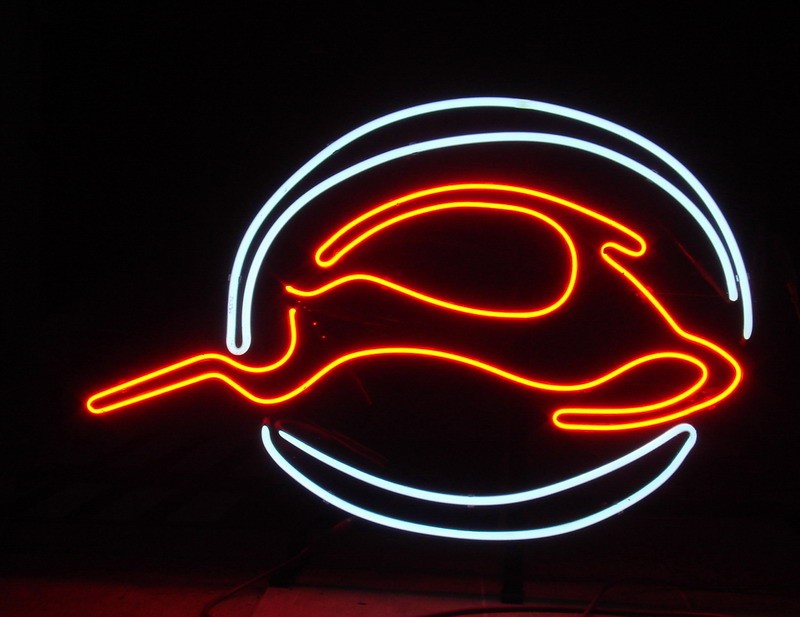A vibrant, full-color photo capturing an indoor neon sign against a predominantly black background, illuminated by artificial light. The bottom of the background reveals a faint reddish tinge, echoing the glow of the neon sign. At the heart of the composition is a striking orange depiction of a running or leaping creature, resembling an elk or antelope with unusually long horns that extend from its head all the way back over its body to its tail. Encompassing this central figure are two sets of gently curved white lines: one set forming a partial arc above and another mimicking a crescent shape below. The interplay of the neon's orange and white hues against the dark backdrop creates a visually arresting and detailed image, evoking a sense of dynamic motion and ethereal illumination.